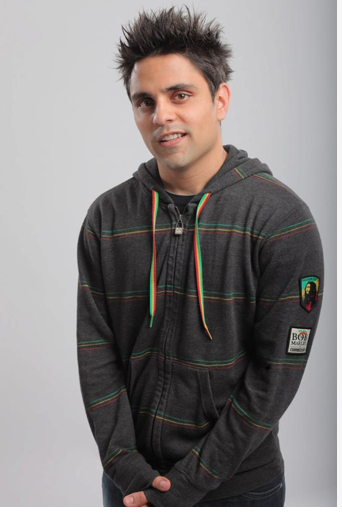The photograph depicts Ray William Johnson, a prominent YouTuber, from the hips upwards. He is facing forward with a direct gaze, and has a subtle smile on his face. His black hair is neatly styled, and he appears to be of Caucasian descent. Ray is wearing a distinctive black zip-up hoodie adorned with occasional green, yellow, and red stripes, which also appear on the pull straps of his hood. Notably, the right sleeve of his hoodie features a patch with Bob Marley's face and another patch at the bottom that reads "Bob Marley." He has both arms positioned in front of him, with his hands casually crossed around his hip. He is paired with blue pants. The background behind him is a gradient gray, lightening towards the center and darkening towards the edges and corners.